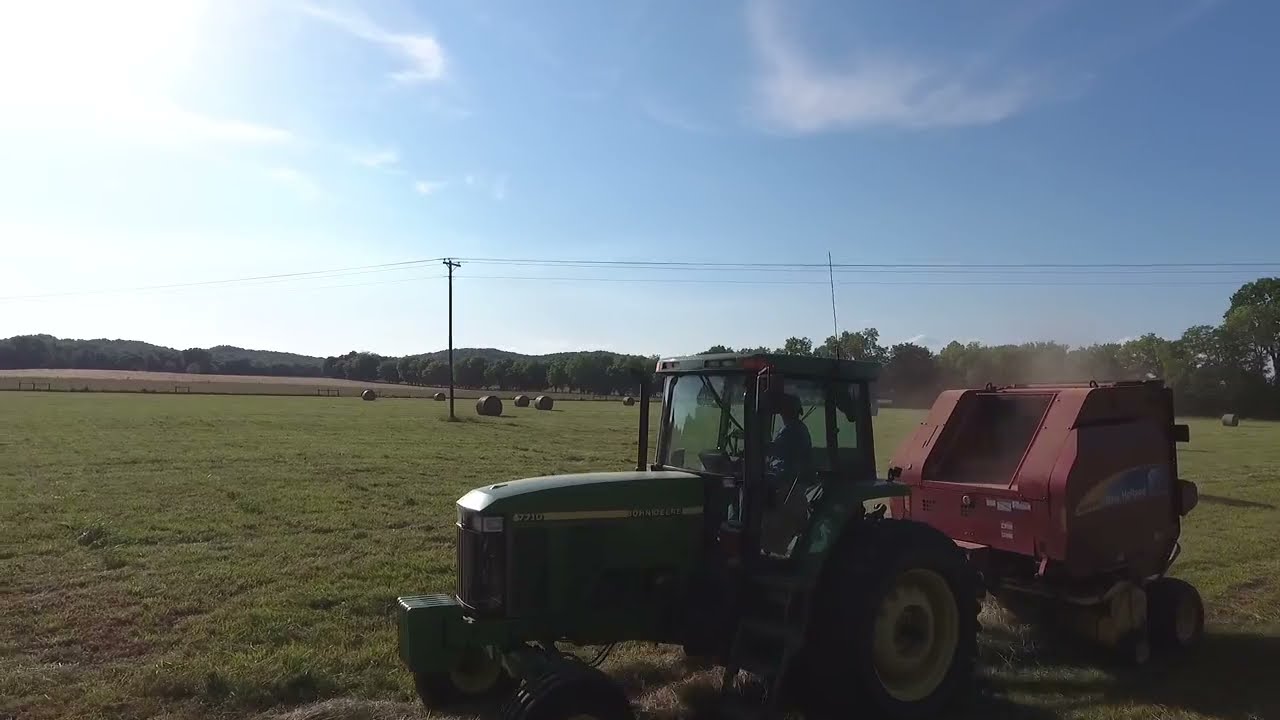The rectangular photograph, oriented horizontally, showcases a scenic farm during the daytime. The top half reveals a stunningly clear blue sky adorned with feathery white clouds and a brilliantly bright sun in the upper left corner. Below, rows of green-leaved trees stretch across the distant middle of the image. The foreground is a vibrant green grass field dotted with bales of hay. Utility poles and lines punctuate the landscape, adding to the rural charm. Centrally positioned at the bottom, a large John Deere model 7710 tractor, resplendent in green with massive black tires and yellow rims, captures attention. Driven by an indistinguishable figure partly visible through the window, the tractor is towing a sizable red apparatus, possibly a wood chipper or a fertilizer spreader. A trail of dust billows from the top of this attachment, adding a dynamic element to the serene farm scene.